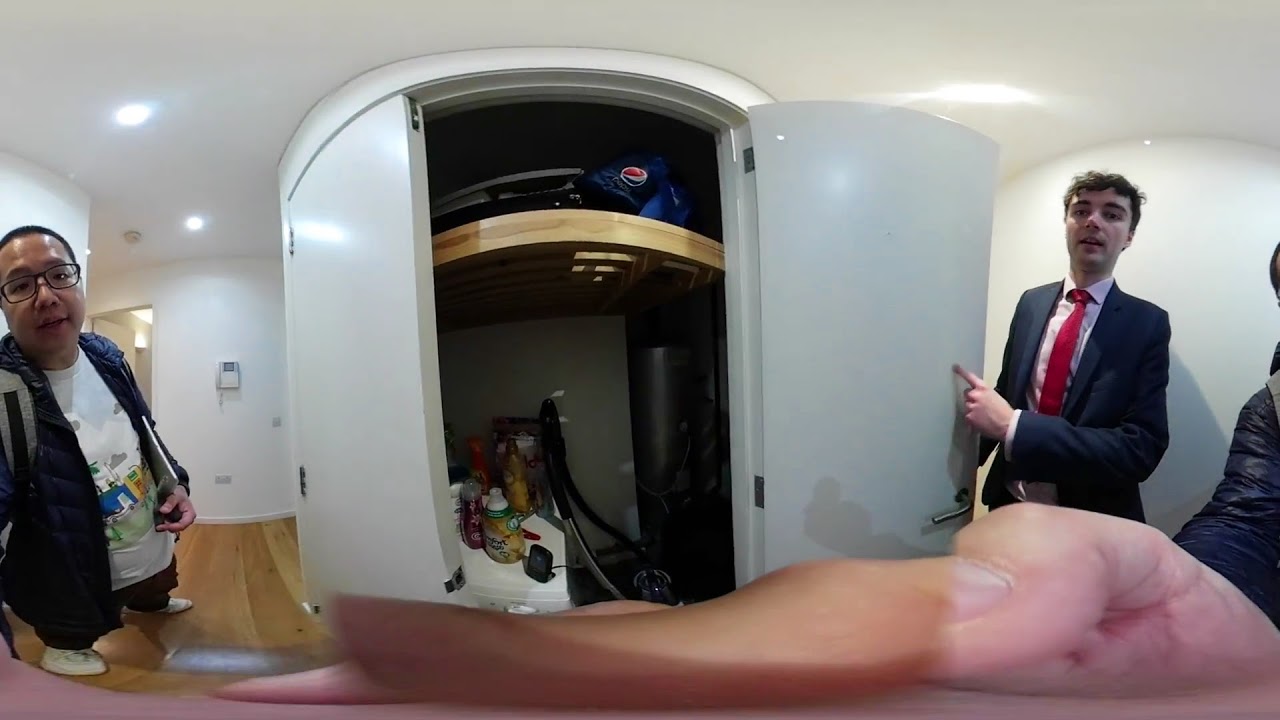An image depicts an interior scene with white walls, a light brown wooden floor, and a white ceiling with two illuminated lights above. Three individuals are present, though the third is partially cropped off on the right side, visible only by a thumb. Predominantly featured are two men: the one on the left of Asian descent, wearing black glasses, a blue jacket over a white shirt with a design, dark jeans, and white shoes, and the other, a tall Caucasian man with curly black hair, dressed in a blue suit jacket, a red tie, and a white shirt. The tall man is opening a white closet door with a silver handle and pointing inside. The closet appears to be a utility storage area containing a washer, dryer, furnace, various detergents in yellow, orange, and purple, and a vacuum with a black hose and silver bottom. There's also a bag stored on the brown wooden shelf inside, adorned with a red, blue, and white logo that resembles a Pepsi design. A telephone, either gray or white, is mounted on one wall, reinforcing the indoor setting of this detailed room.